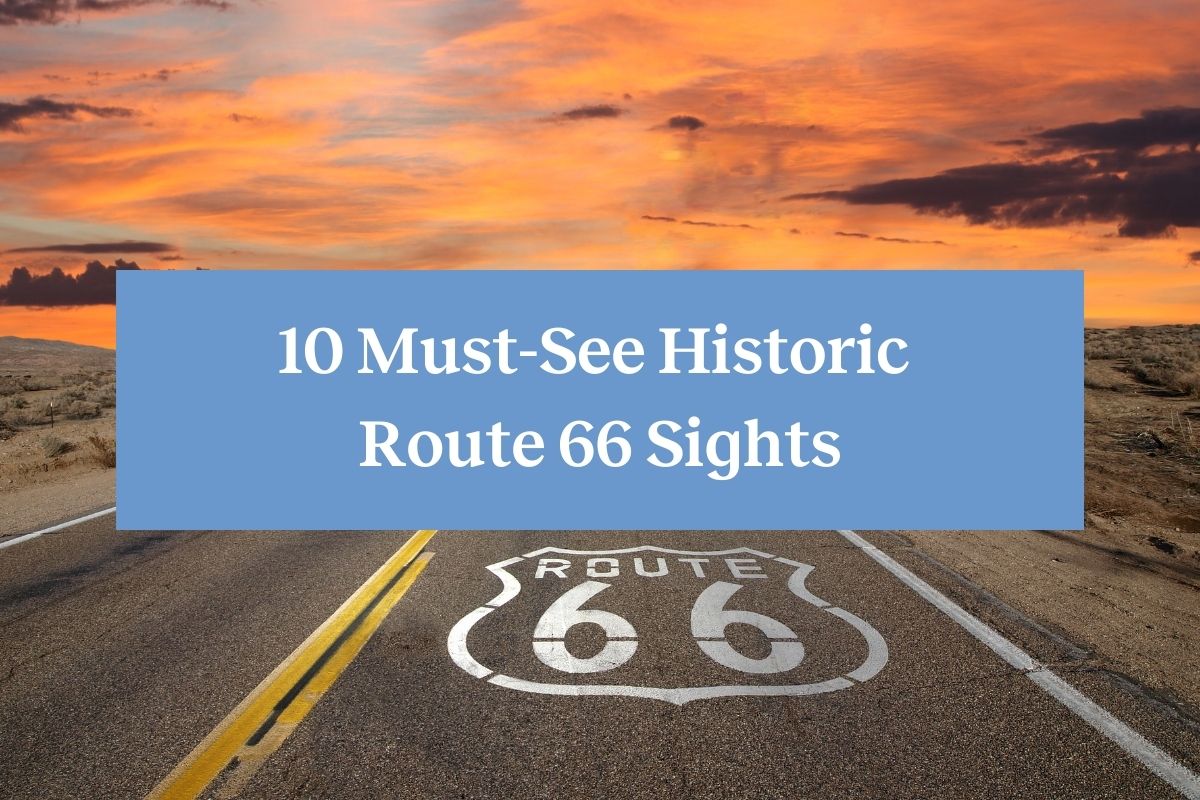The image depicts a desert landscape with Route 66 prominently featured on the road. The road is marked with a distinctive shield emblem, indicating "Route 66" etched onto the pavement, likely added digitally. The highway has a yellow center divider and white lines on both edges, designating it as a two-lane road. The surrounding landscape is arid and shrub-filled with a hill on the left side. The sky above is a striking blend of amber and orange hues, reminiscent of a sunset. Overlaid on the image is a light blue rectangular block of text. In bold white letters, it reads "10 must-see historic Route 66 sites," with "10 must-see historic" on the top line and "Route 66 sites" beneath it. The overlay is conspicuous, drawing attention to the informational content about Route 66 attractions.